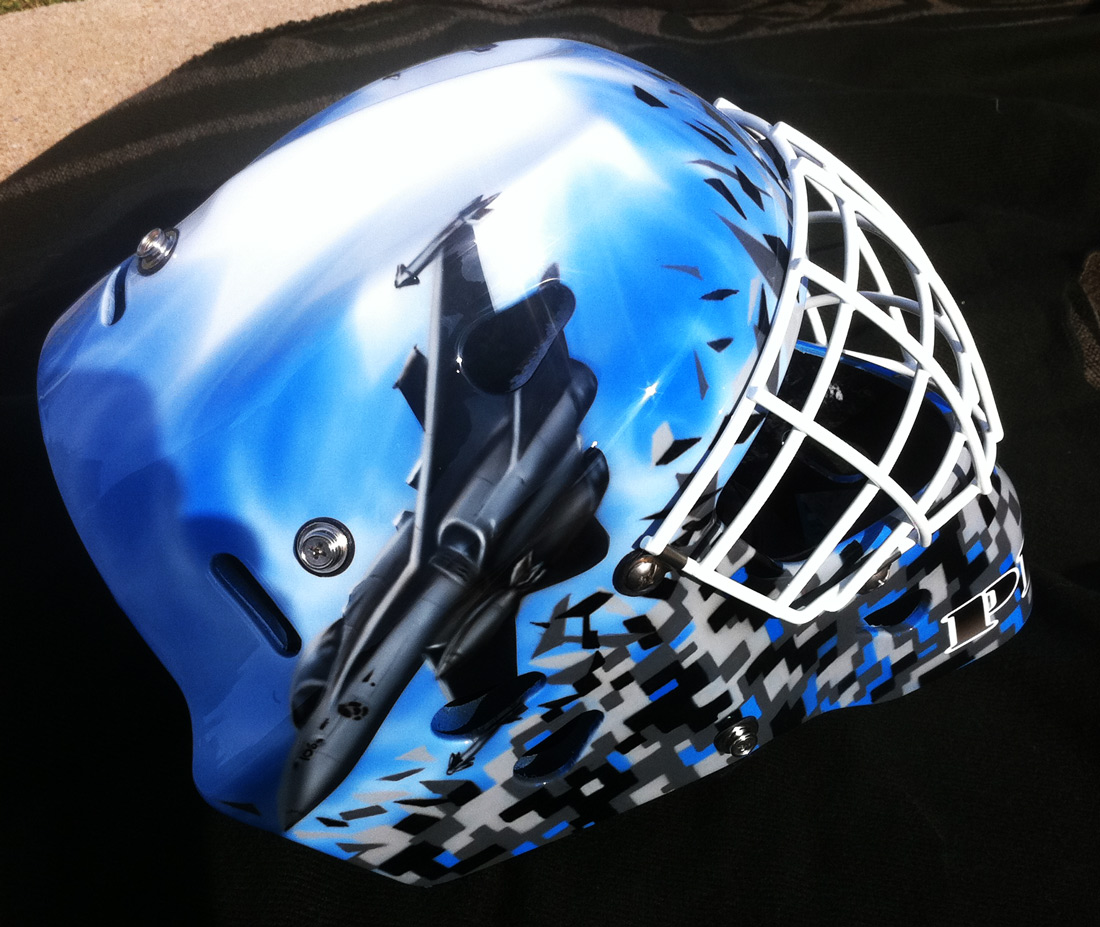The image features a hockey helmet resting on a black fabric with subtle gray stripes, set against a small visible corner of a tan-colored rug. The helmet has a distinctive design with a white face mask, consisting of a gridded cage-like structure, located in the upper right corner of the image. The helmet's color palette includes various shades of blue, light gray, dark gray, and black, similar to small pixel-like shapes scattered around its surface. A prominent feature of the helmet is a detailed depiction of a military jet, oriented towards the back and appearing to fly downward and leftward, with missile-like projectiles on its wings. Additionally, there's a partial word near the front starting with the letter 'P', though the rest is cut off. The helmet's positioning on the black fabric with the rugged background details suggests it's being displayed carefully and deliberately.